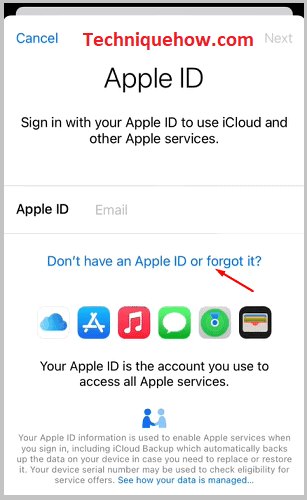**Screenshot Caption:**

This image is a detailed screenshot from an iPhone, specifically showcasing an Apple ID sign-in screen. Dominating the view is the Apple ID interface, which prompts the user to "Sign in with your Apple ID to use iCloud and other Apple services." 

At the top of the screen, in blue text, is the "Cancel" option, followed by a red "technique.com" link and a "Next" button in light gray. Below the title "Apple ID," another prompt is seen in dark black, along with a field labeled "Email" in light gray.

In blue text, there is a link stating, "Don't have an Apple ID or forgot it." A series of six small icons representing different colored iPhones (blue, red, green, white, and black) follow. The black icon, located furthest to the right, features a red arrow pointing to the "Forgot" link at the top.

Further details explain the significance of an Apple ID: "Your Apple ID is the account you use to access all Apple services." Adjacent to this text are two figures illustrated in blue. Additionally, the text clarifies that the Apple ID information enables various services, including the iCloud backup, which helps preserve your device's data for replacement or restoration purposes. It also notes that the device's serial number may be used to check service eligibility and manage data usage.